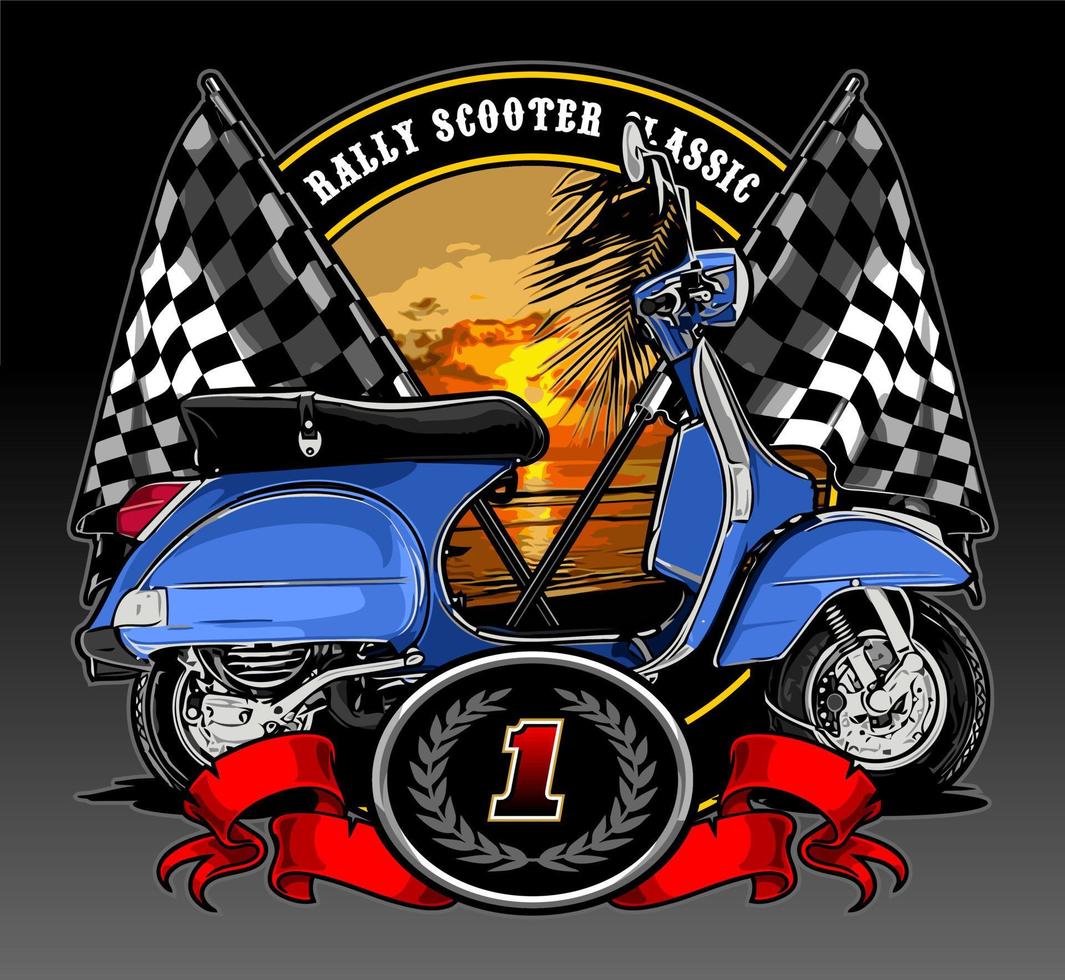The image is an animated or digitally illustrated scene featuring a blue scooter with a black leather seat and rear-view mirrors. It has a classic and polished look, including a headlight and fully aired tires. The background transitions from dark black at the top to gray at the bottom. At the top of the image, there's a prominent black banner outlined in yellow, displaying the text "Raleigh Scooter Classic" in large white capital letters. Directly below this text, a colorful sunset scene in shades of orange and yellow serves as a scenic backdrop. Two crossed black-and-white checkered flags lean outward from the scooter, enhancing the racing theme. In front of the flags and taking center stage is the side view of the blue scooter facing right. On the front of the scooter, a circular emblem boasts a bold red "1," surrounded by silver leaves and accented with a red ribbon swirling around the circular outline. A shadow is visible near the scooter’s tires, adding depth to the illustration.